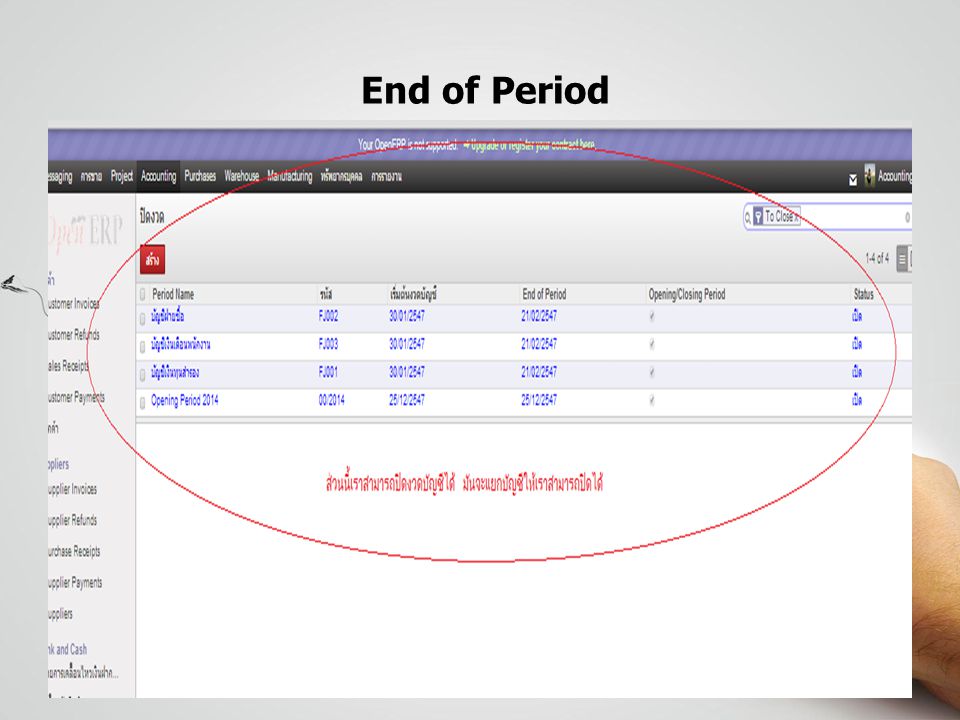The image shows a PowerPoint slide featuring a screenshot of project management software. At the top of the slide, a bold black header reads "End of Period." Below this, there is a blue banner and a gray sub-header, with a dynamic background featuring lighter gray and white elements, possibly including an indistinct arm graphic.

The central part of the slide displays a screenshot of a computer application, structured in a table format with multiple columns and rows. Column titles include "Period Name," "End of Period," "Opening," "Closing Period," and "Status." Within these columns, there are four rows of blue text. This central area of the screenshot is encircled by a red oval, likely drawn using Microsoft Paint, with additional red text that is difficult to discern. The blue text in the screenshot appears to indicate various dates and status information, with an overlay of red lettering that might resemble Thai script.

Additional design elements include a small red icon on the top left of the screenshot, a blue top border containing white and green text, and a black border at the bottom right featuring a profile image beside the word "Accounting." This descriptive detail emphasizes the structured and informative nature of the slide while highlighting the key visual elements shared across the different descriptions.